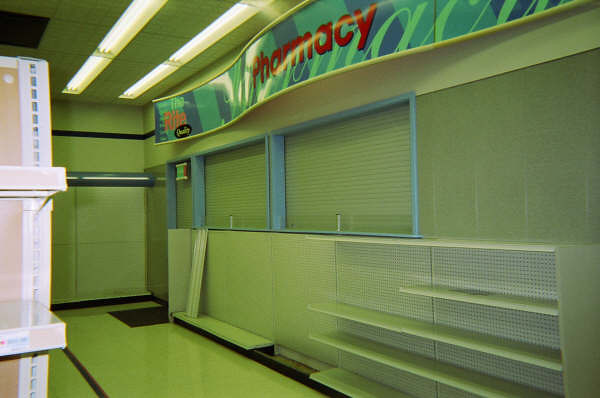This image captures the interior of a store, specifically focusing on the pharmacy section. The scene features a prominent sign overhead with the word "Pharmacy" written in bold red letters. The front of the pharmacy is closed off with a roll-down security shutter covering the windows. The shelving units are completely barren, devoid of any products, contributing to an overall atmosphere suggesting the store is not currently in operation.

The ceiling is lined with about eight fluorescent light fixtures, all of which are illuminated, casting reflections onto the pharmacy sign below. This sign is notably long and features a distinctive wavy design with blue and darker blue striping. The window frames of the pharmacy are painted in light blue, adding a subtle touch of color to the otherwise minimalistic scene.

The walls, shelves, and floor are predominantly white, although the floors and walls appear slightly yellowed, possibly from age or the lighting. This detailed composition conveys an ambiance of emptiness and closure within the store's pharmacy section.